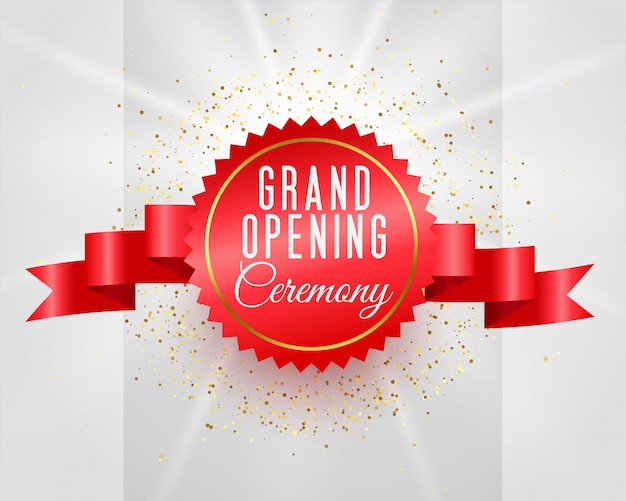The image features a vibrant red ribbon with a pronounced circular centerpiece that conveys a celebratory theme. The ribbon, extending horizontally to both the left and right, has distinctive V-shaped cutouts at its ends. At the center of the ribbon, there is a prominent red circle adorned with pointed star-like edges, encircled by a gold border. The inner part of the circle contains the text "GRAND OPENING" in bold white capital letters, with "CEREMONY" written in elegant white cursive underneath.

The backdrop is primarily a light gray gradient, transitioning to a darker gray at the center behind the ribbon. This area is further embellished with an array of tiny, colorful dots, primarily in gold and bronze hues, which radiate outward from the red circle. Additionally, white rays emanate from the circle, extending both upwards and downwards, adding a dynamic sparkling effect. The combination of the intricate ribbon design, the celebratory text, and the shimmering background creates a festive and elegant visual.